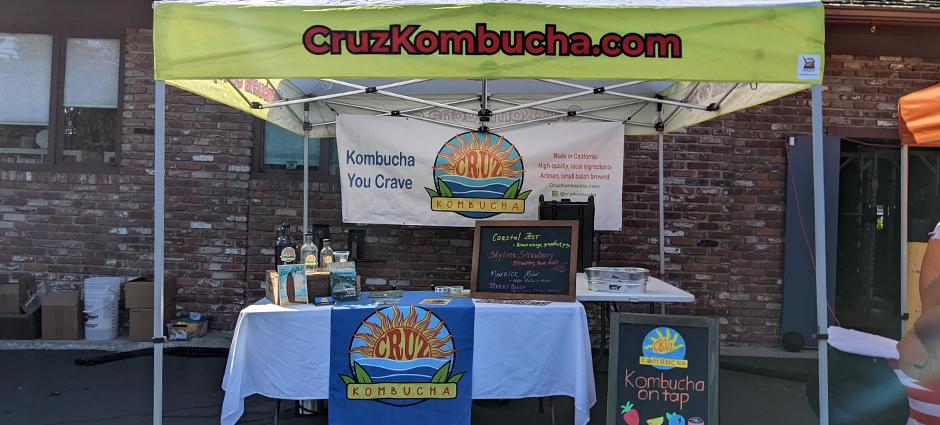The photograph captures an outdoor scene at a likely farmers market or craft fair, featuring a bright and organized kombucha stand under a pop-up tent from CruiseKombucha.com. The tent structure is silver with a yellow top, prominently displaying the company's website in bold red letters. At the center of the setup, a long table is draped with a white tablecloth and additional branded fabric showcasing the company logo—a sun over waves with leaves and a yellow banner stating 'Kombucha.' Various bottles of kombucha are neatly arranged on the table, emphasizing the range of products for sale. A small, colorful chalkboard menu is positioned on the right side, although its text remains unreadable in the image. Behind the table, a white banner reads "Kombucha You Crave," reinforcing the branding. The setting includes a background that features a red brick building with windows framed in brown and fitted with white shades, adding to the warm, community-oriented atmosphere of the event.